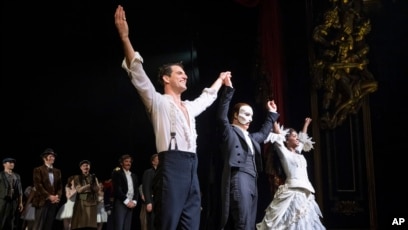The photograph captures a scene from a likely stage production of "Phantom of the Opera." Three main characters are prominently positioned at the front of the stage, holding their hands up in what seems to be a triumphant gesture, possibly taking a bow after a performance. The man in the center, presumably portraying the Phantom, wears a white mask and a dark blue suit with a white shirt. To his left is a woman dressed in a vintage white dress with a corset adorned with frills, and to his right, a man in an old-fashioned white shirt, blue pants, and suspenders. The scene appears to be set indoors, with other actors visible in the background, though their details are obscured by distance. The rectangular photograph includes the initials "AP" in white at the bottom right corner, potentially indicating it was distributed by the Associated Press.